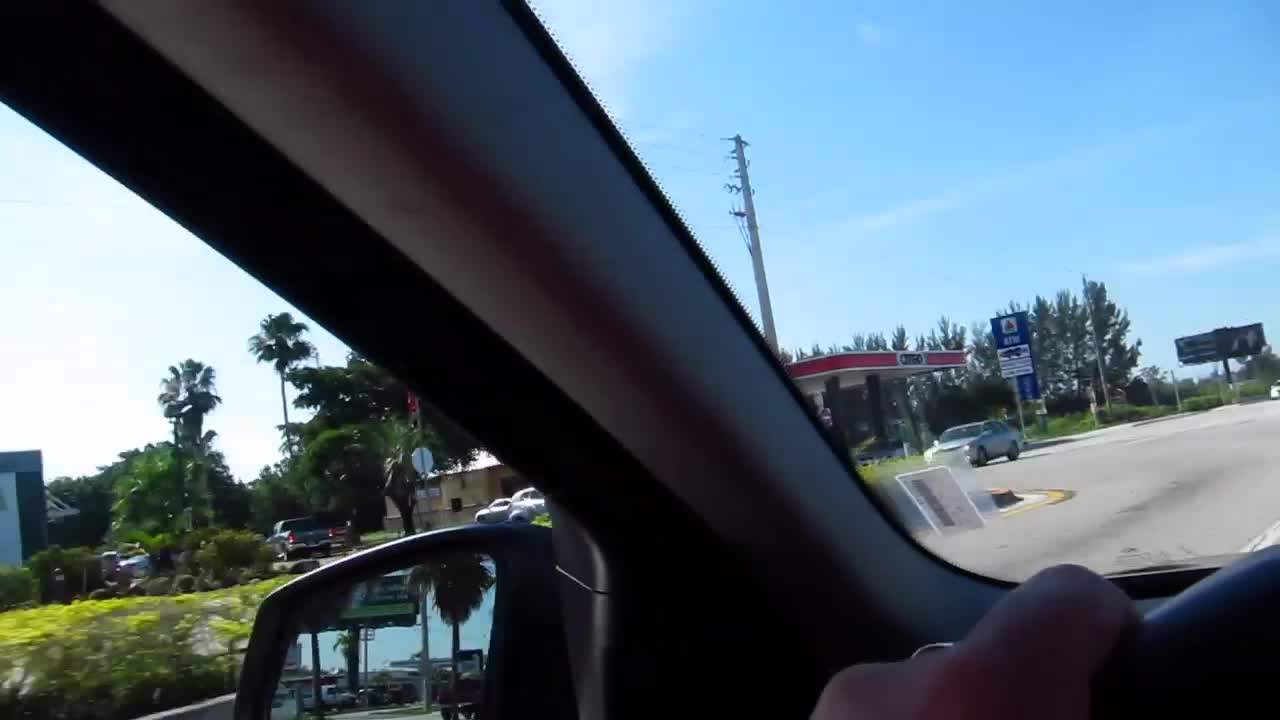This photograph, oriented horizontally, captures the viewpoint of a person driving a car with the steering wheel positioned on the left side, indicating a left-hand drive vehicle. The image includes a wide-angle view of the interior and exterior environment: the lower right corner reveals the driver's hands gripping the steering wheel, while the left section of the frame showcases the road as seen through the windshield and the driver's side window.

Prominently, a gas station with the Citgo logo is situated ahead and slightly to the left, visible through the windshield. A vehicle is parked at this station. The rearview mirror in the lower center of the photograph reflects additional scenery, including several palm trees, suggesting a warm climate setting. Further in the background, a line of trees, comprising more palm trees and other types, stretches behind the gas station and along the left side of the frame. A highway sign appears ahead, indicating the presence of a structured roadway network. The combination of these elements clearly places the scene in a sun-soaked, possibly coastal region with typical tropical or subtropical vegetation.